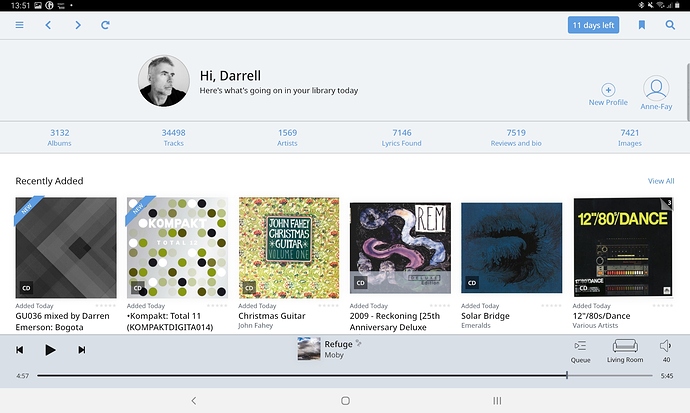The image features a detailed user interface. At the top, there is a black strip displaying the time as 13:51. Below it, a gray area contains three horizontal lines on the upper left side, representing a menu icon. To the right of these lines are navigation buttons: a left arrow for 'back', a right arrow for 'forward', and a refresh button. Next to these is a prominent blue button labeled "11 days left" and a magnifying glass icon for search functionality.

On the far right of this gray area, there is a black and white round profile picture of a user, possibly named Daryl. Below this gray section, a text message reads, "Hi Daryl, here's what's going on in your library today."

Further down, a detailed breakdown of the library's contents is presented with the following statistics: 
- New Profile: Anne Faye
- 3132 albums
- 34,498 tracks
- 1,569 artists
- 7,146 lyrics found
- 7,519 reviews and bios
- 7,421 images

Following this informational text, a "Recently Added" section features six different album covers. The first album on the left is titled "GU-036 mixed by Darren Emerson, Bogota." The album next to it is "Compact Total 11, Compact Digital 014." The third album displayed is "Christmas Guitar."